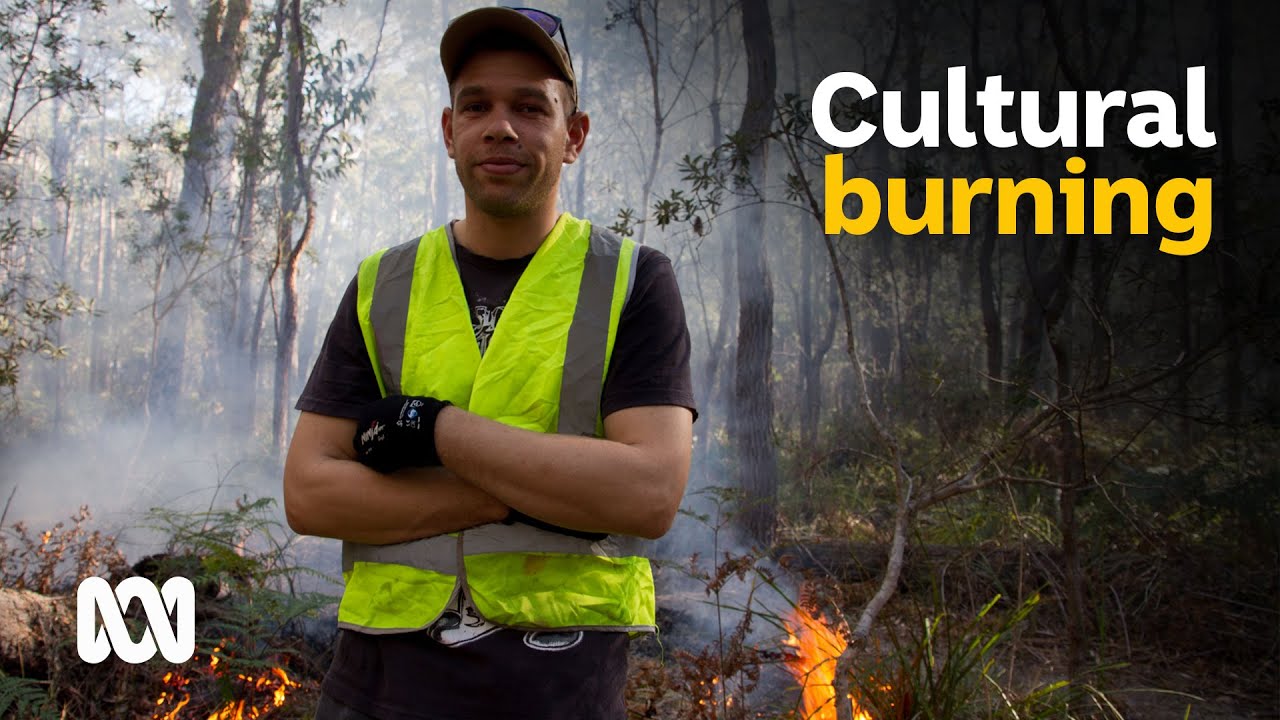A vibrant, color photograph in landscape orientation captures a man standing slightly left of the center in front of a burning forest. The man, exhibiting a calm demeanor with a light smile, has dark skin and is visible from head to mid-hip. He wears a bright yellow-green safety vest with gray stripes, paired with a black short-sleeved t-shirt, black gloves, and black pants. His brown cap is pulled up over his forehead, with sunglasses resting atop it. The man's arms are folded across his chest, adding to his composed appearance.

Behind him, flames consume shrubs and ground cover on both the right and left sides, emitting smoke that slightly obscures the moderately bare trees in the background. The fire likely represents a controlled cultural burn, although the specifics are unclear from the image alone.

In the upper right corner, the words "cultural" in large white letters and "burning" in gold letters stand out prominently. The lower left corner features a triangular logo consisting of interconnected white lines, adding a subtle graphic element to the photograph. The overall style of the image is realistic, emphasizing the detailed scene and the man’s poised presence amidst the controlled blaze.